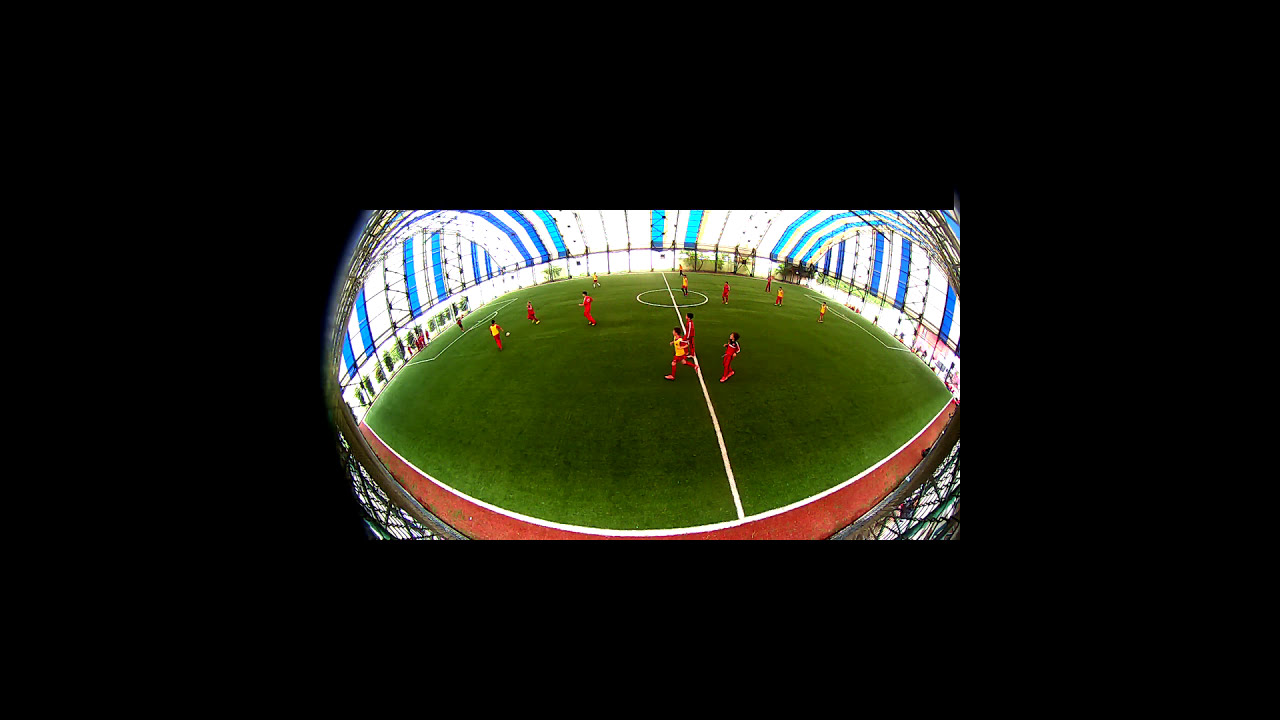The image captures an indoor arena taken from an elevated perspective, revealing a circular field with a distinct, dark border framing the photograph. The center field is lush green, segmented by white lines and a central circle, suggesting it is a sports field. Scattered across the field are eleven players, most donned in red jerseys with hints of yellow attire, appearing to be engaged in a game, possibly soccer given the presence of marked goals on either end. The arena's perimeter features a white interior barrier resembling a fence, and beyond it, the walls display blue arches with vertical blue lines ascending. The arena's dome-like, enclosed structure suggests it is an indoor facility, with the vivid colors of black, brown, green, tan, white, red, yellow, and light blue vividly contrasting against the surrounding darker frame.